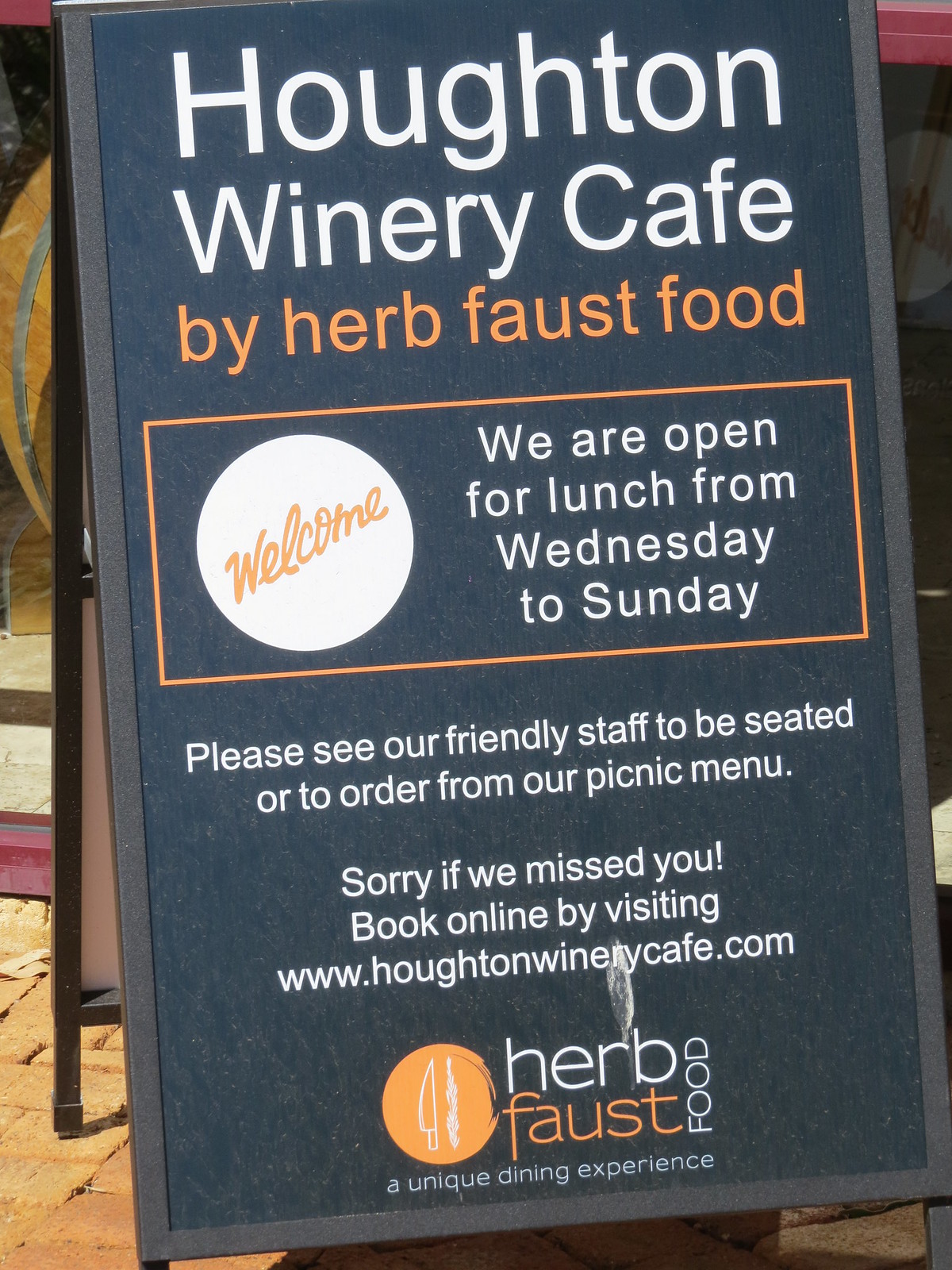The image depicts a professionally designed, fold-out advertising sign positioned outside the Houghton Winery Cafe. The prominent two-sided board, mostly blue, features multiple sections with key information. At the top, "Houghton Winery Cafe" is displayed in bold white letters. Below, in vibrant orange, "Buy Herb Faust Food" is written in lowercase. An eye-catching white circle on the left side contains the word "Welcome" in orange cursive, slanted from the bottom left to the top right. Accompanying text on the blue background announces that the cafe is open for lunch from Wednesday to Sunday. Further down, an orange rectangular box asks patrons to see the friendly staff for seating or picnic menu orders and provides an apology with booking information, directing visitors to book online at www.houghtonwinerycafe.com. At the very bottom, against an orange circle, a sharp knife and another tool in white lines frame the tagline, "Herb Faust Food, a unique dining experience." The scene is set in daylight, casting a slight shadow on the sign's legs, indicating late afternoon or early evening hours, with no people visible in the image.